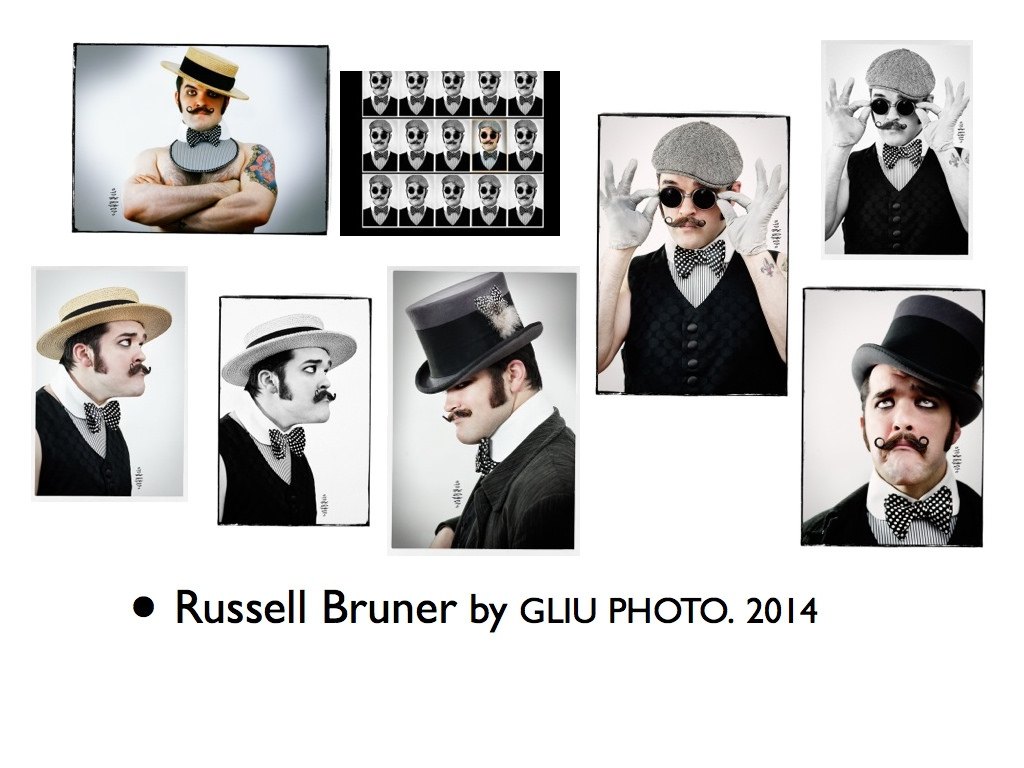This image showcases a series of eight small photographs on a white background, prominently featuring a man named Russell Bruner, as highlighted by the caption "Russell Bruner by GLIUphoto2014" at the bottom center. Each photograph displays Bruner in various old-timey, throwback outfits with a modern or edgy twist. He has dark hair, long sideburns, and a distinctive handlebar mustache, with some images showing the mustache's edges twirled up. Bruner is adorned in different headwear, including top hats, flat straw hats, and beret-type hats. His attire across the photos features a mix of vests, large black and white bow ties, and other vintage-inspired fashion elements. One notable photograph includes him wearing a hat, a bow tie, a bib, but no shirt, revealing a muscular build and a large tattoo on his shoulder. These photographs capture Bruner in various poses from the waist up, accentuating his carnival owner-esque style reminiscent of depictions from the 1930s and 40s.